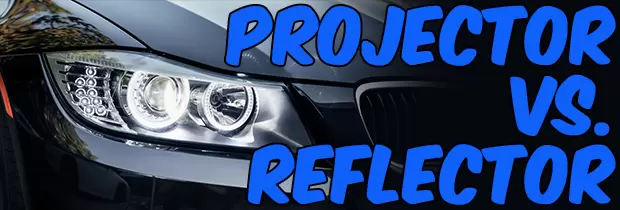This image features a glossy black car prominently displaying its front left side, with a clear emphasis on its headlight area. The headlight, adorned with an acrylic cover, showcases two distinct lamps and is encircled by smaller elements. Reflections of trees can be seen on the car's shiny surface. Spanning the right side of the image, vibrant blue slanted text that reads "Projector VS. Reflector" in a fun, rounded font with a black outline dominates the background. The placement and style of the text suggest it might be part of an advertisement or a promotional graphic, potentially discussing different types of car headlights. On the left-hand side of the image, you can observe parts of the car's hood, grille, and a hint of orange peeking through, all gradually fading into a deep black on the right.